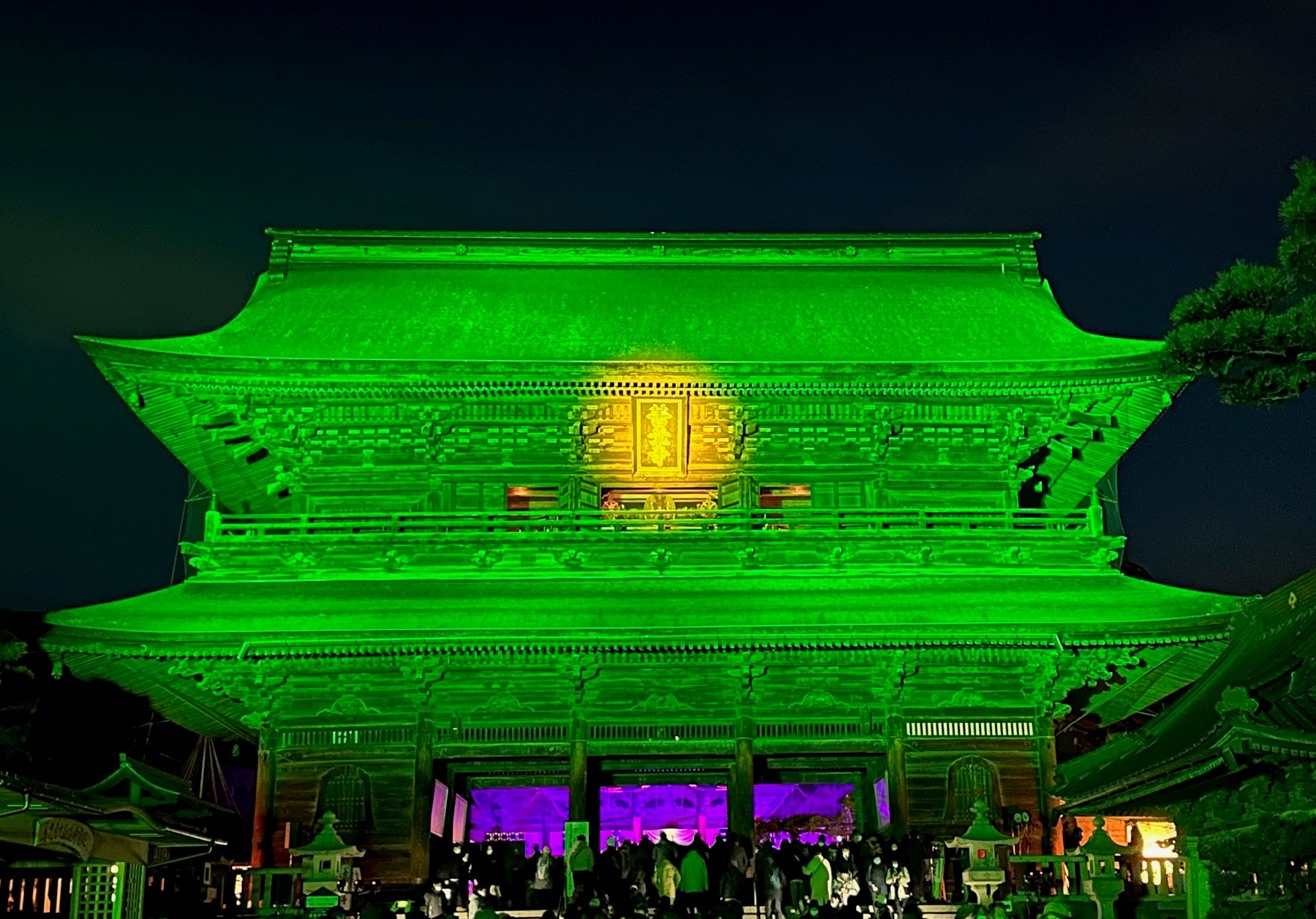A vibrant, neon-lit Chinese architectural marvel stands prominently in an evening or nighttime setting. The structure, reminiscent of ancient Chinese styles, is bathed in radiant lime green light, accentuated by a central yellow circle on the two-tiered roof. The dark background sky enhances the vivid luminosity of the building, which also displays purple lights within its interior, especially under the first tier. Numerous tiny, shadowy figures congregate around the structure, suggesting a bustling crowd. To the building's right side is a neon-green tree, while additional green-lit buildings and vegetation fill the scene. The overall effect is as if viewed through night vision gear, adding an otherworldly ambiance to the photograph.